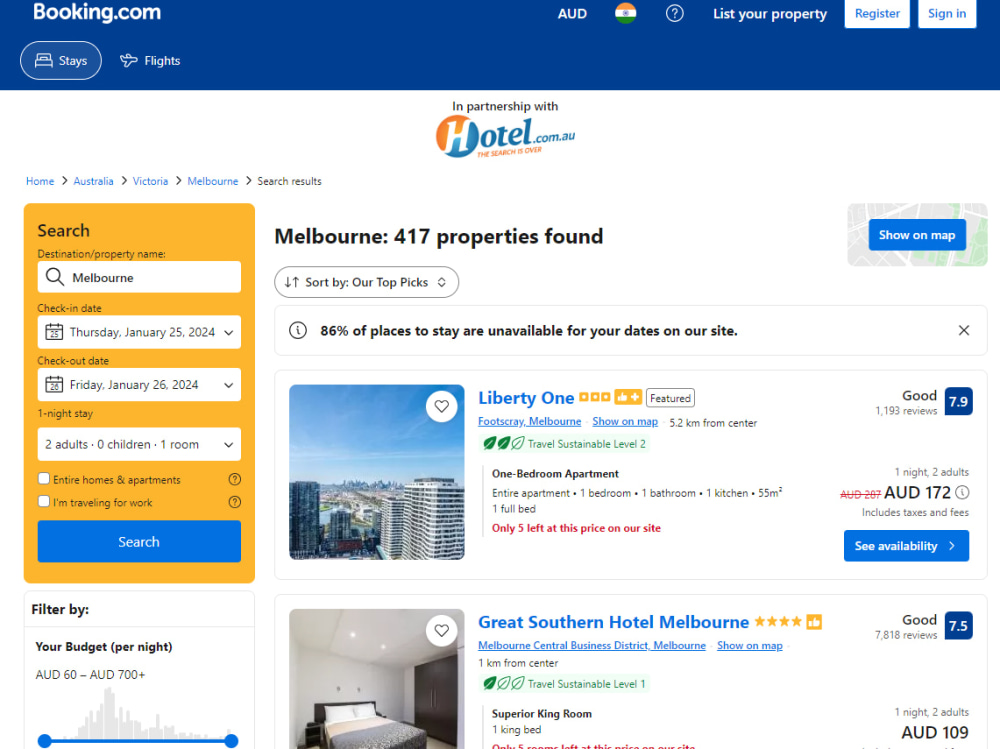The image is a screenshot from the booking platform called Booking.com. At the top of the page, there's a prominent blue rectangle stretching across the entire width. Along the left side, there's a search area designed in a yellowish-orange hue. The central section features multiple images, providing a visual representation of different options. At the top of the middle section, there are tabs for switching between "Stays" and "Flights". The header displays "USD" next to a flag icon within a circle, a question mark within a circle, and links to "List your property", "Register", and "Sign in".

Amid the page content, there’s a banner indicating a partnership with Hotels.com.au. There is also a highlighted destination, "Melbourne", which notes that 417 properties were found. Users can sort these properties by "Our top picks". It’s mentioned that 86% of places to stay are unavailable for the selected dates on the site.

As you scroll down, specific properties are listed including "Liberty 1" and the "Great Southern Hotel Melbourne". For each property, there are details about its star rating, guest reviews, pricing, and additional information.